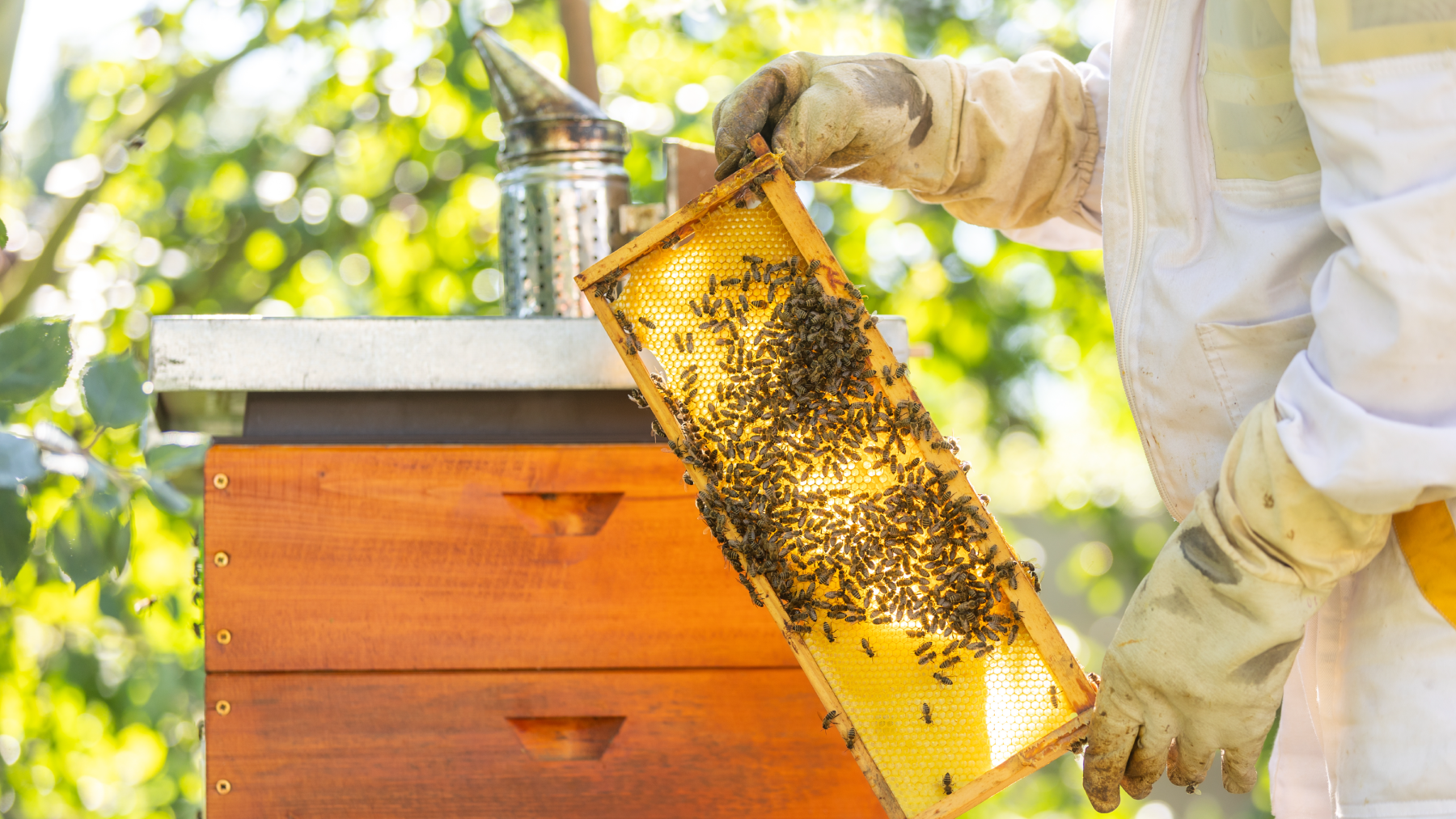In the sunny outdoor setting of a lush, green-leafed garden, a beekeeper clad in a full white protective suit, including gloves stained with black marks, is visible from the neck down on the right side of the image. The beekeeper is attentively holding a yellow honeycomb rack brimming with bees. Positioned in the center of the scene is a weathered wooden beehive with a natural wood texture and a white top. Atop the beehive sits a smoker, resembling an oil can, used to calm the bees with smoke. The background reveals a blurry yet discernible array of green and yellow leaves, suggesting a tranquil, sun-dappled day.